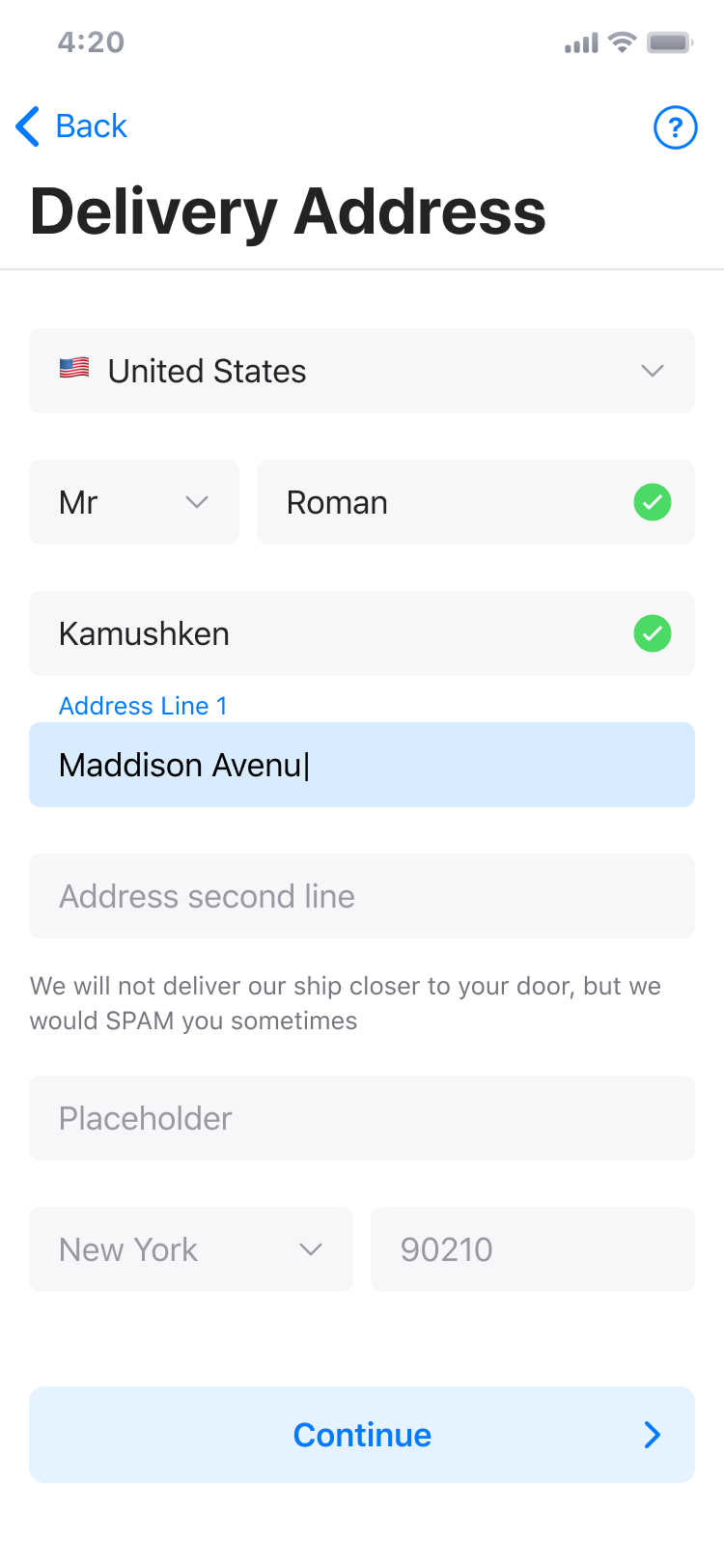A screenshot of a cell phone display featuring a detailed delivery address form. At the top, the status bar displays the time as 4:20, alongside icons for network coverage, Wi-Fi connectivity, and battery level. Below the status bar, there is a navigation pane with a blue left arrow labeled "Back" and a blue question mark inside a blue circle for help or information. The section titled "Delivery Address" specifies the destination country as "United States," addressed to "Mr. Roman Kamushkin," with the family name spelled out as "K-A-M-U-S-H-K-I-N." The address continues with "Address Line 1" set as "Madison Avenue," while "Address Line 2" remains unspecified. A message indicates that delivery services will not bring shipments directly to the door but may occasionally send spam. The placeholder for the address is "New York, 90210." The bottom of the form includes a blue "Continue" button for progressing to the next step. The image is entirely text-based, with no photographic elements or visual depictions of people, animals, plants, buildings, or vehicles. The overall orientation of the screenshot is vertical, being taller than it is wide.